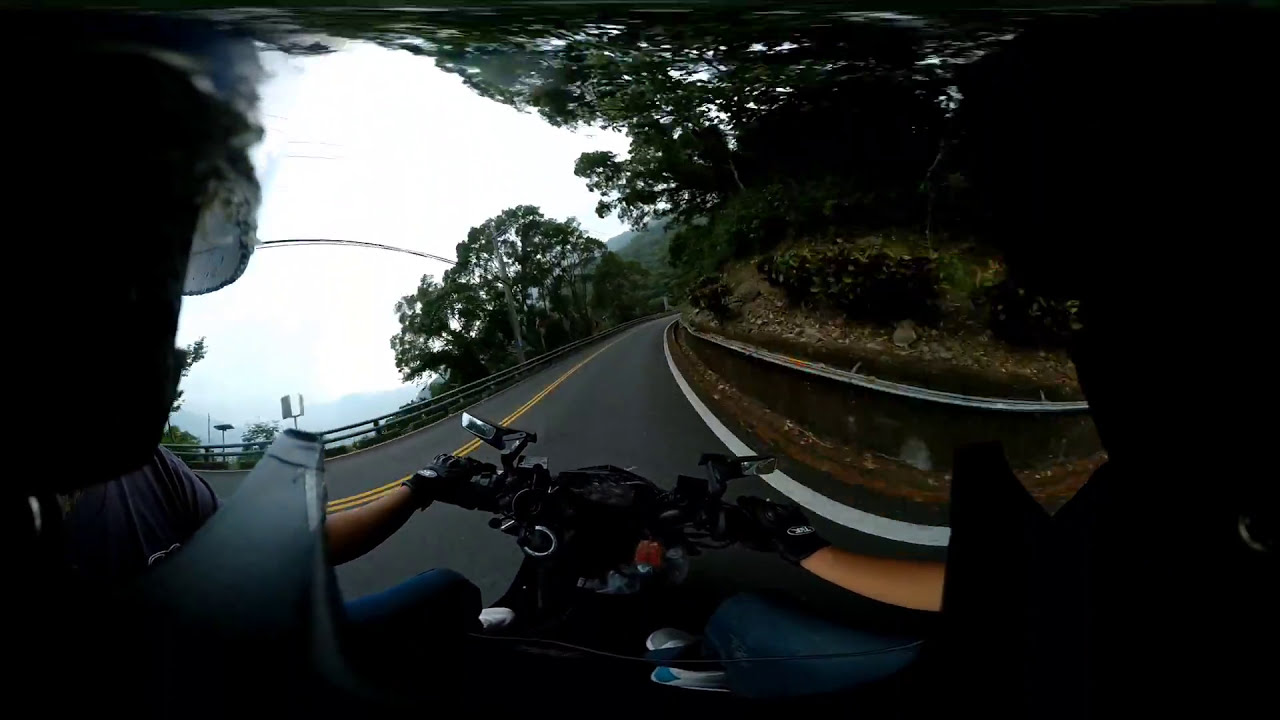This horizontal photograph captures a motorcyclist riding along a winding mountain road. The perspective suggests it’s taken from slightly behind and to the side of the rider, who is adorned in casual attire including jeans and likely gloves, with a watch visible on the left wrist. On the left side of the image, the road is bordered by a steep drop-off with a protective railing, descending sharply to a canyon with visible trees and mountains in the distance. The right side showcases the hillside with a curved curb running along the road, leading to a sloping terrain that descends towards water at the bottom. Flanking the road on both sides are dense trees, with branches stretching across the top of the image, implying an overhead canopy. Additionally, power lines can be seen above the road, all under what seems to be a clear daytime sky.